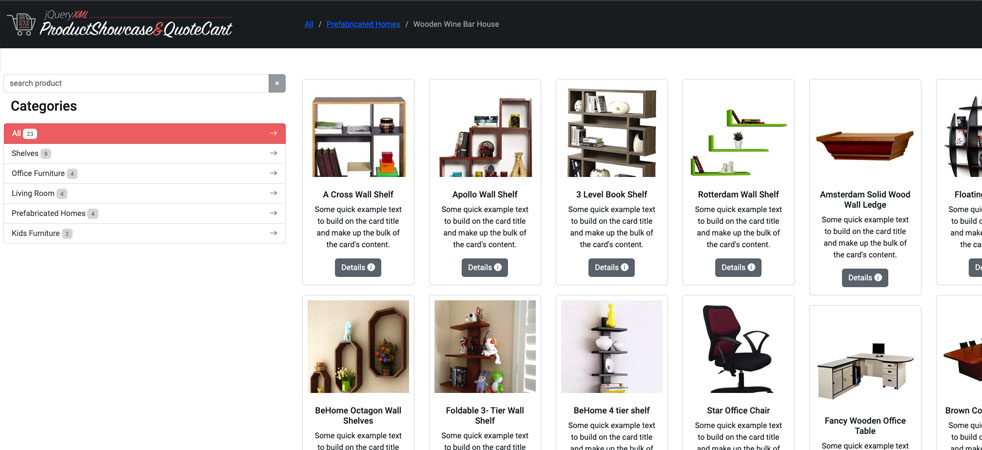**Caption:**

The top banner features a sleek black background. On the left side, in white text, it says "Product Showcase" followed by "Cart" twice. Blue and gray fonts are used to the right of this section. Below the banner, the categories are listed, followed by an orange box and some tiny gray lettering at the bottom. A gray arrow on the right side points towards the right.

The main display consists of a grid of product images, arranged with six images per row. Each product is presented on a white background with black lettering.

**First Row:**
1. "Across Wall Shelf" in black text with a "Details" button in a gray box featuring white lettering.
2. "Apollo Wall Shelf" with black text in the middle and a "Details" button at the bottom.
3. "Three-Level Bookshelf" with small text detailing the product, and a "Details" button underneath.
4. "Rotterdam Wall Shelf" with a "Details" button.
5. "Amsterdam Solid Wood Wall Ledge" with a "Details" button.
6. The last image in this row appears to be cut in half.

**Second Row:**
1. "Behome Octagon Wall Shelves."
2. "Foldable Three-Tier Wall Shelf."
3. "Behome Four-Tier Shelf."
4. "Star Office Chair."
5. "Fancy Wooden Office Table."
6. The final image in this row is partially cut off and shows a brown color.

This detailed layout provides a comprehensive view of the available products, making navigation easy for users.